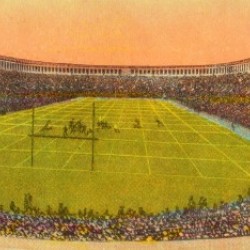This image is a detailed, vintage-style illustration of a football field viewed from one of the end zones. The sky is a vibrant coral pink, adding an unusual yet striking background to the scene. The field itself is a bright lime green, marked with white grid lines that stretch into the distance. The end zone features traditional goalposts forming a U-shape. Surrounding the field is a stadium packed with spectators, depicted as little dots to indicate a full house. The stadium consists of a single tier of seating that envelops the field, with a distinctive horseshoe shape and upper stone structure with multiple windows, topped by a reddish roof. The illustration also includes players on the field, though they are somewhat vague and indistinct, enhancing the image's vintage and slightly faded quality.